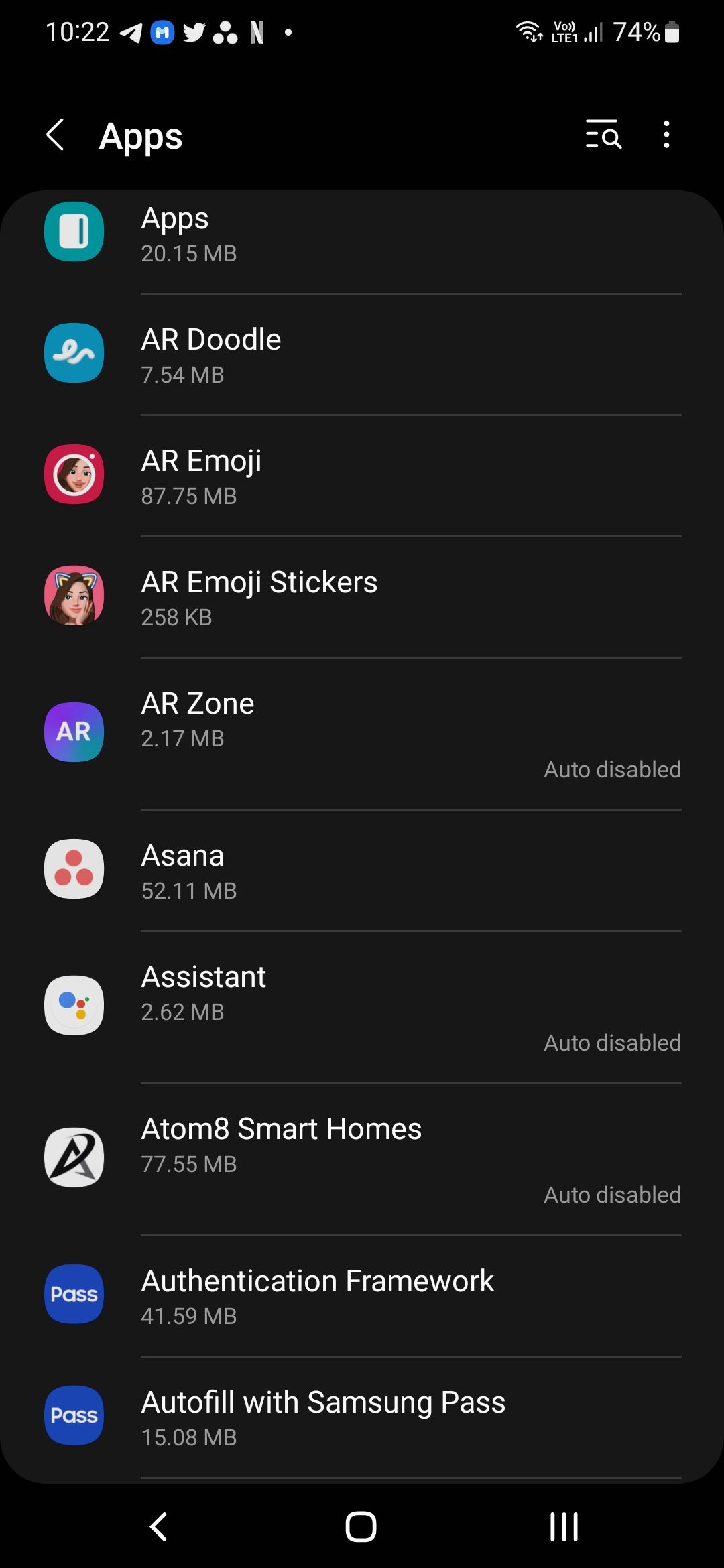The image is a detailed screenshot from an Android phone displaying the "Settings" menu within the "Apps" section. The top portion of the screen features a black background with white text, reading "1022." Alongside this text, there are several app icons: a paper airplane icon, a white "M" on a blue background, the Twitter logo, a triangle of three white circles, the Netflix logo, and a white dot. To the far right, status indicators display a Wi-Fi symbol, LTE symbol, cellular network symbol, and a battery icon showing 74% charge.

At the bottom of the screen, also set against a black background, there are three simplified white icons for navigation: a back arrow, a home symbol, and a recent apps icon represented by a square, circle, and a rectangle respectively.

In the main section of the screen, there is a white title bar with a back button and the text "Apps" on the left. On the right side of this title bar are three vertical dots, three horizontal lines, and a search icon. Below, a middle section displays a list of installed apps against a grey background with white text detailing each app. The list reads as follows: "Apps, AR Doodle, AR Emoji, AR Emoji Stickers, AR Zone, Asana, Assistant, Atom 8 Smart Homes, Authentication Framework, Autofill with Samsung Pass." Each app entry includes the app's name in bold white text, its logo to the left, and the app size in smaller text beneath the name.